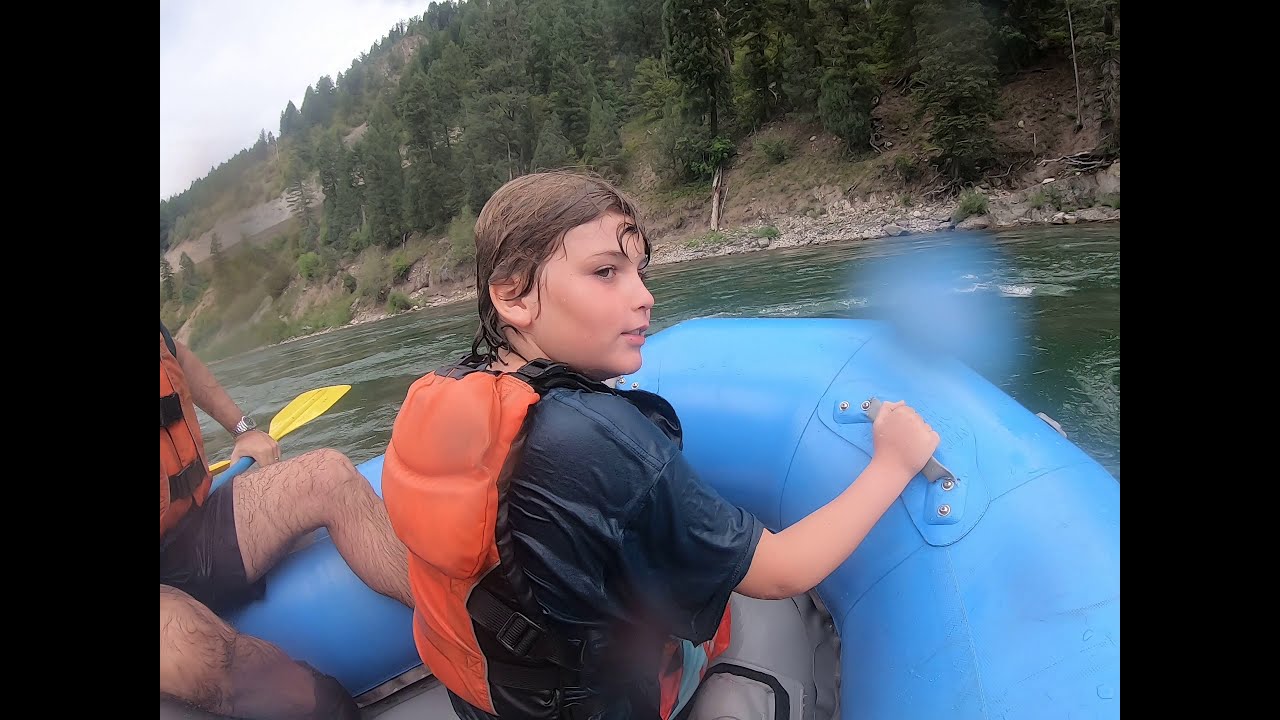The image captures a scenic outdoor moment of a river rafting adventure. Set against a picturesque backdrop of forest green waters and a mountainous range densely populated with pine trees, a bright blue inflatable raft navigates the river. Inside the raft, a soaked young boy with wet brown hair dons a black shirt and an orange life vest, gripping a handle for support. Beside him is a partially visible man wearing soaked black shorts, also equipped with an orange life vest, and wielding a blue and yellow paddle. Both appear content and immersed in their adventurous activity. The surrounding landscape includes rocky outcrops and lush greenery, with water droplets splashed on the camera lens, enhancing the dynamic and refreshing environment.